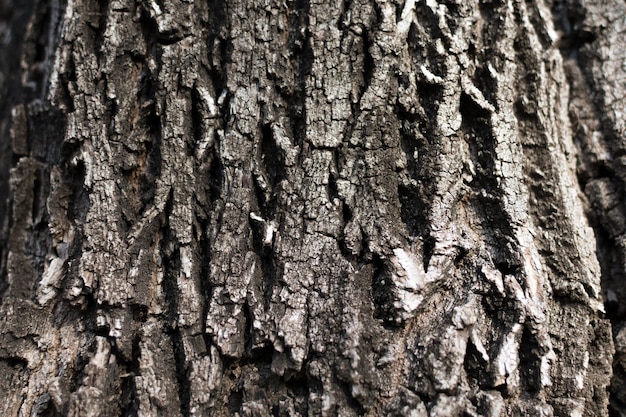This close-up image captures a detailed segment of tree bark, revealing a textured, vertical orientation of overlapping, layered strips. The bark, characterized by its dark brown and gray hues with intermittent white patches—possibly highlights from sunlight—appears robust and healthy, devoid of peeling. The intricate bark structure includes at least eight vertical stripes with underlying gaps. The surface looks rough and scraggly, implying a sharp texture to the touch. Despite being part of a larger trunk, the image focuses narrowly on this fragmented section, showcasing the tree’s rugged exterior without any visible branches or leaves. The photograph itself is of low resolution.